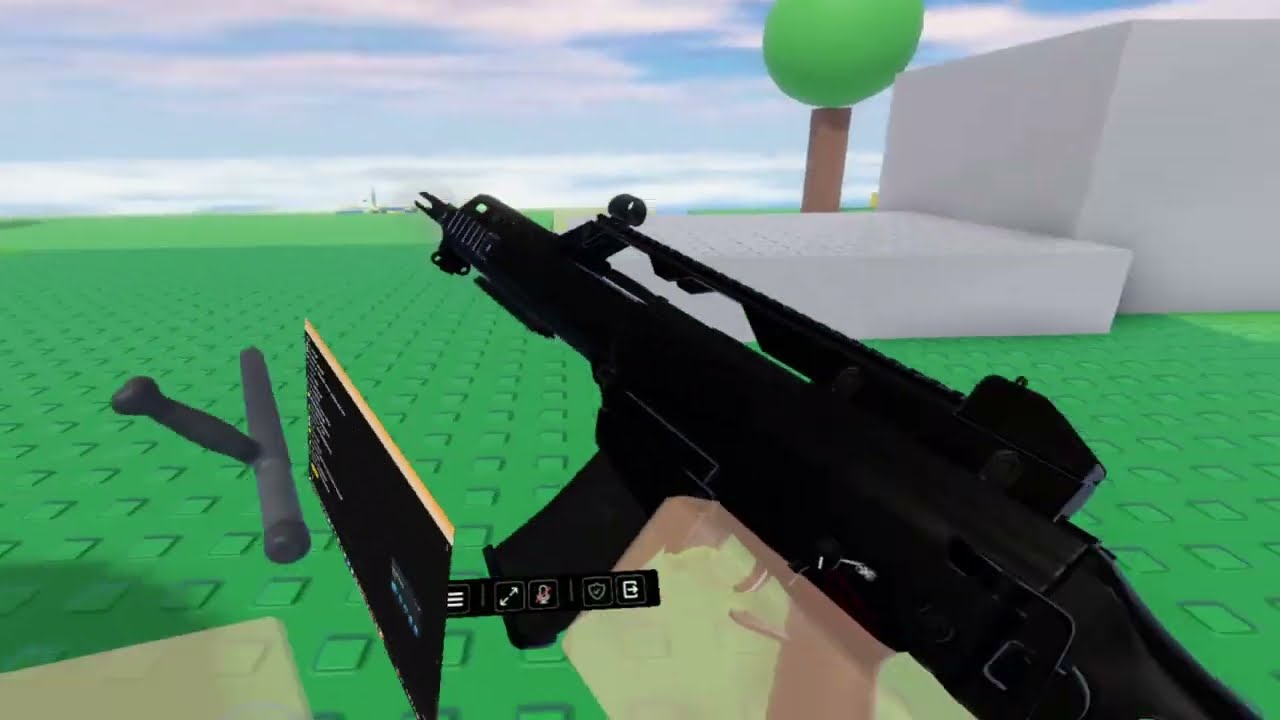The image is a highly pixelated screenshot from a first-person shooter video game, potentially a sandbox-style game such as Gary's Mod, Minecraft, or Roblox. The player's perspective shows them holding a black automatic rifle with a scope. The ground consists of green, Lego-like blocks. To the left below the gun, there appears to be a web computer screen or frame, possibly indicating game controls or a design element. On the right side of the view, there are two small grey squares forming a platform and a larger grey square resembling a building. A rudimentary tree, composed of a vertical brown pole topped with a circular green shape, stands in front of these squares. Scattered white cubes and various other seemingly out-of-place objects can also be seen in the background. The sky is depicted as blue and cloudy, adding a more immersive element to the game's environment.